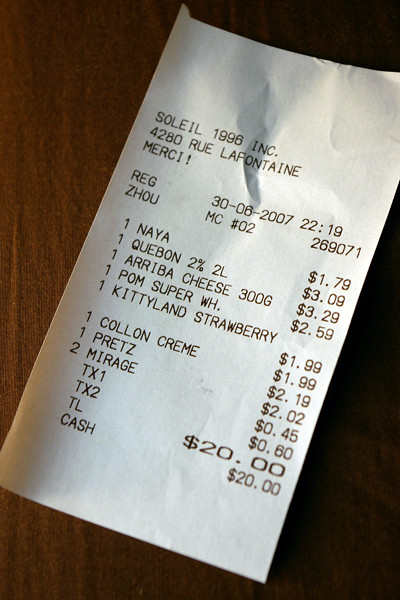Close-up image of a white receipt laying on a wooden table. The receipt is oriented at an angle, with the bottom left corner pointing slightly to the left and the top right corner tilted to the right. The top of the receipt prominently displays "SOLEIL 1996" in ink, followed by a street address listed as "4280 Rue LaFontaine." Below the address, the word "MERCI!" is printed, conveying a thank you message to the customer. The receipt shows a total amount of $20, which was paid in cash.